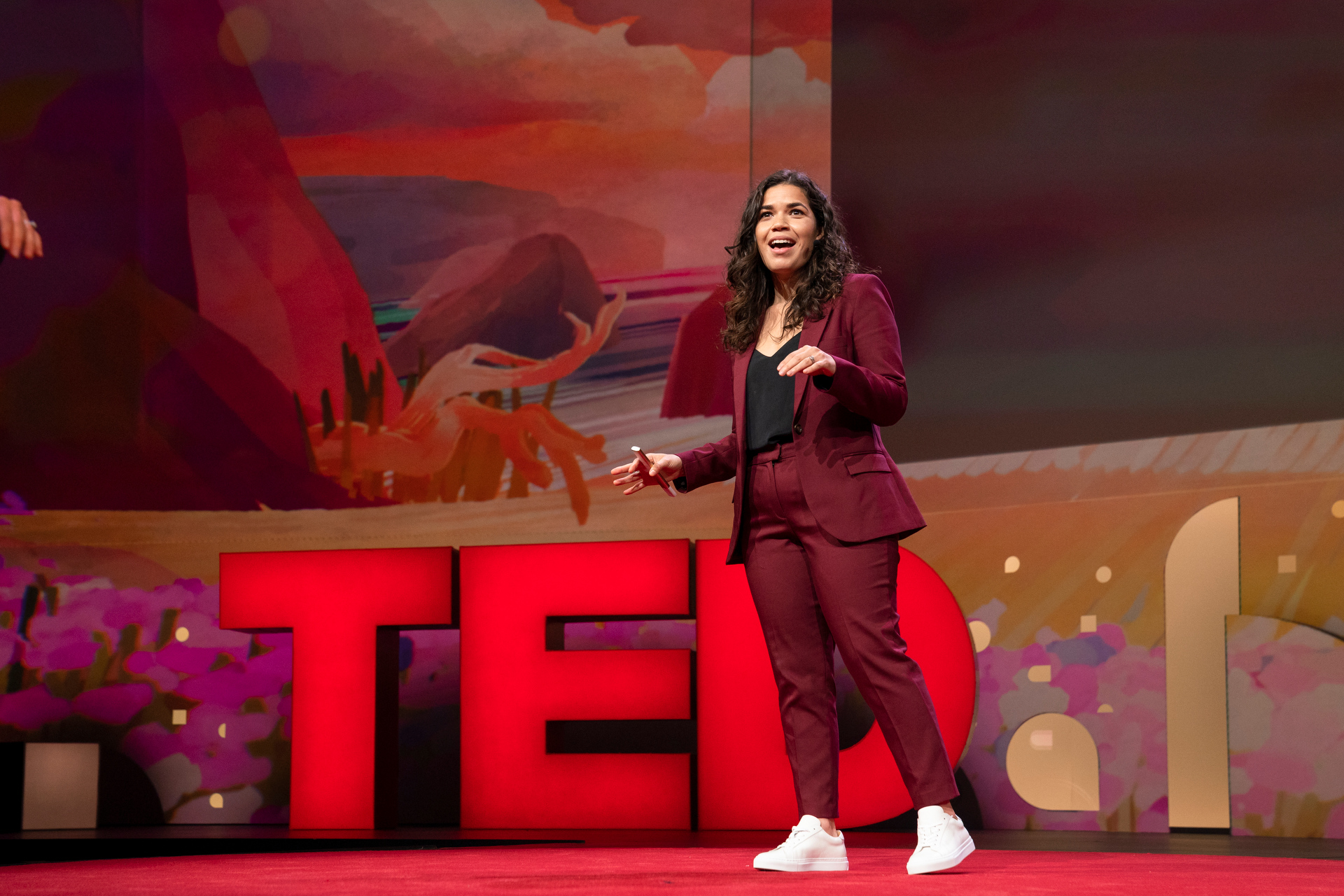The image is a vibrant color photograph capturing a Latina actress, possibly America Ferrera, delivering a TED talk. She stands confidently on a pinkish-red carpeted stage, almost centered in the frame, with giant, physical letters spelling "TED" beside her. The backdrop features an intricate seascape artwork with rocks, water, clouds, and an array of colorful elements, including variations of red, orange, purple, and blue. The actress is dressed in a coordinated maroon blazer and matching pants, paired with a black, low-cut V-neck tank top and bright white sneakers. Her long, curly brown hair cascades down as she appears to be mid-speech, fully engaged with her audience. Judging by the high quality of the photograph, it seems likely to have been captured by a professional photographer or paparazzi.